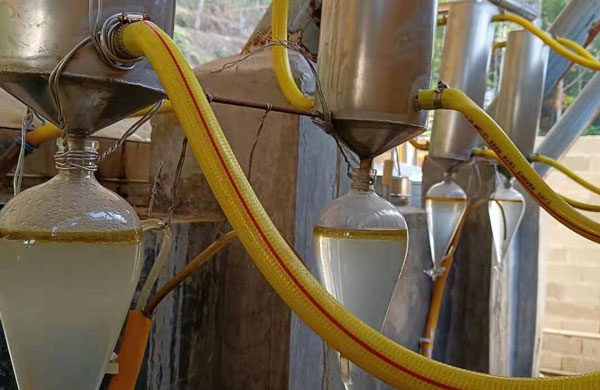The image depicts a landscape-oriented setup, possibly a distillery, featuring a neat row of identical apparatuses. Each unit consists of a silver canister at the top and a teardrop-shaped glass bottle at the bottom, held together with wire. Bright yellow hoses are connected to both the top and bottom of the canisters, suggesting a system where some substance, potentially air, gas, or liquid, is being fed in or out. These units are aligned next to each other, mounted on a concrete post. Within the glass bottles, there is a clear liquid with a yellowish film on top, along with visible condensation. The pointed end of the teardrop-shaped glass bottles faces downward, each fitted with a small spigot for dispensing the liquid.